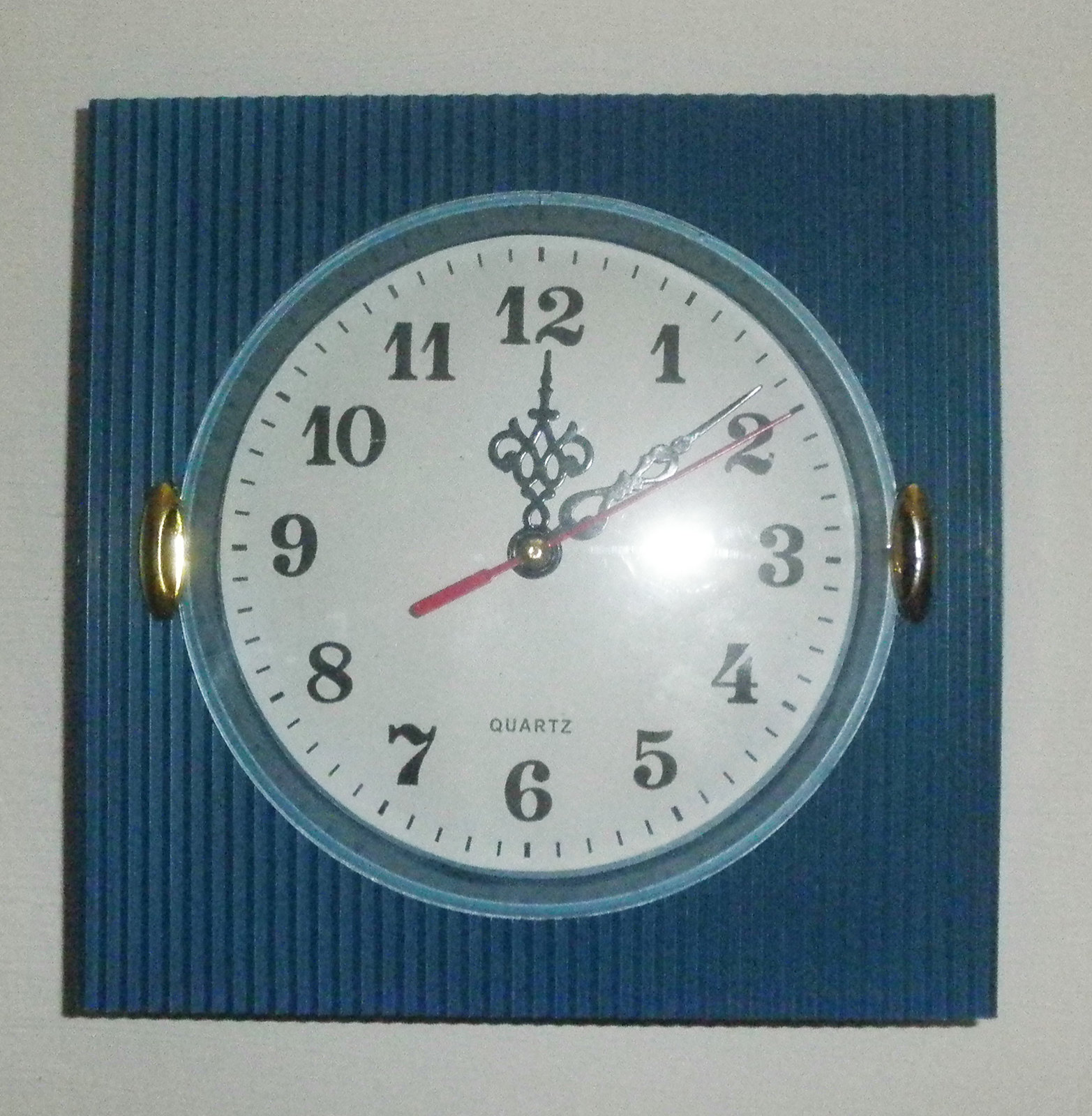The image features an intricately designed timepiece set against a blue backdrop. The timepiece is enclosed in a glass-like case, revealing its detailed inner structure. It prominently displays black numerals and minute markers on the dial, while a distinctive red second hand adds a touch of contrast. The word "Quartz" is inscribed on the face of the clock. On either side of the timepiece, there are gold-toned components, likely serving as winding mechanisms or for similar functions. The clock is placed on a gray surface, though it's ambiguous whether this is part of the clock's design or simply the background on which it rests. The actual size of the clock remains unclear, as there are no reference points to determine whether it is a miniature clock or a full-sized wall clock.